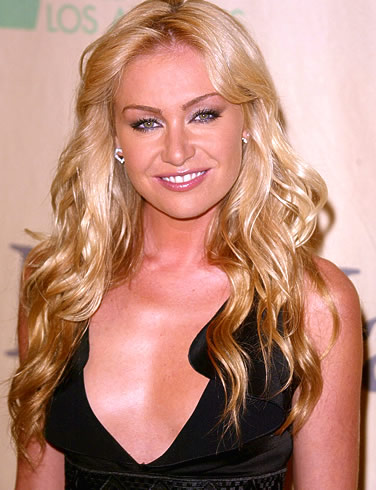The image features Portia de Rossi smiling directly at the camera at what appears to be a red carpet event. She has long, wavy blonde hair cascading far below her shoulders. Her light blue eyes are accentuated by her arched eyebrows, and she's showing her top row of teeth as she smiles. Portia is adorned with diamond heart-shaped earrings, although her right earring is partly obscured by her hair. She is wearing a sleeveless black dress with a wide V-neck. Behind her, the backdrop is a pinkish-gray wall with partially visible text reading "LOS," which likely spells out "Los Angeles," along with other advertising and sponsor logos that aren't fully legible. The setting is bright, with Portia standing against this textured background, slightly angled and poised for the photograph.